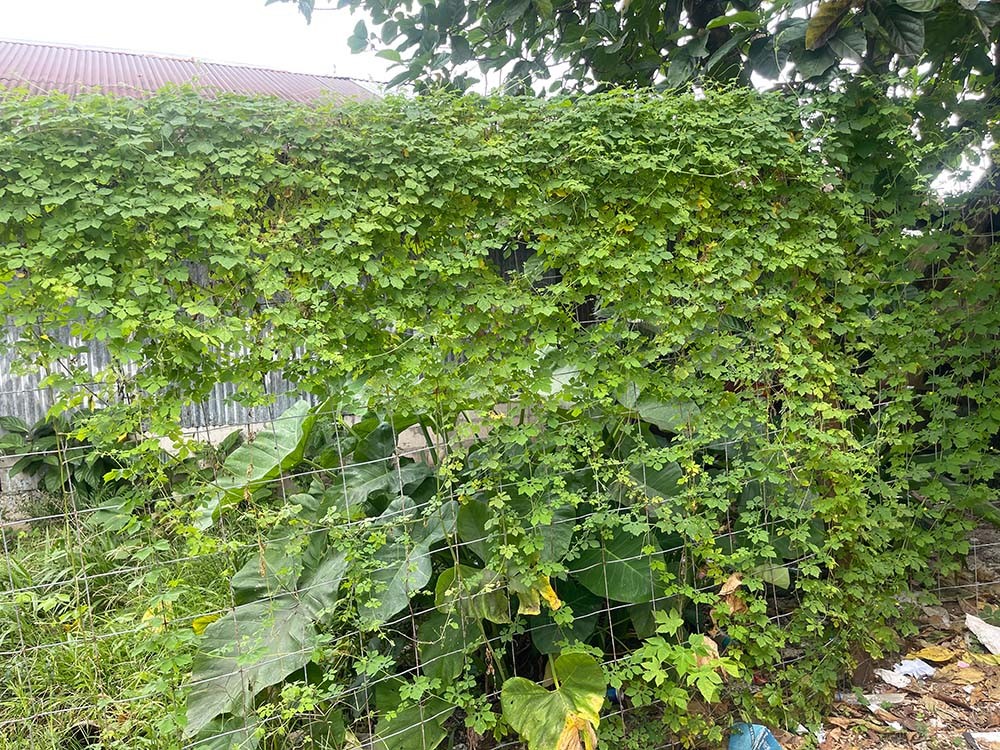This landscape photograph captures an outdoor scene focused on a metal mesh fence with chain-linked squares. The fence, spanning from the left to the right side of the image and almost reaching the top, is adorned with lush green vines, most of which cluster thickly at the top, obscuring much of the fence. The lower part of the fence remains more transparent due to fewer vines. Behind the fence, various large, leafy plants, including some with leaves significantly larger than the vine leaves, are visible along with patches of grass.

In the background to the left, a large corrugated metal building with a triangular red roof adds an industrial touch to the scene. The structure’s rusty, silver-gray sides contrast with the greenery. Above and to the right of the building, the top of a leafy deciduous tree peeks into the frame, set against a hazy white sky.

In the bottom right corner of the image, the foreground features some brown debris—comprising leaves, sticks, and potentially some garbage—lying in front of the fence. Overall, the image embodies a photographic representational realism style, presenting a grounded, detailed view of the naturally and human-maintained environment.